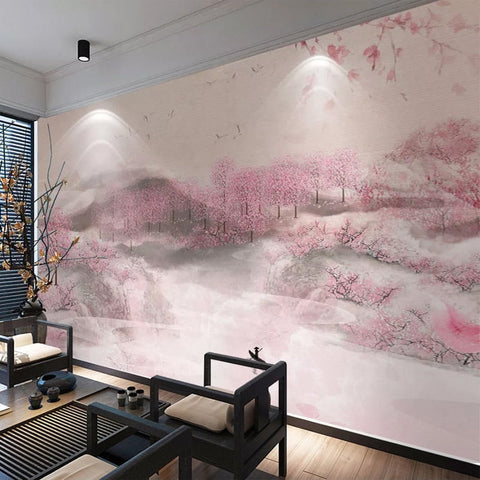The image depicts a modern room with sleek design elements, possibly a living room or a waiting area. The walls are a crisp white, creating a clean and airy atmosphere. The floor is made of wood, enhancing the room’s warm ambiance. Central to the room are two stylish black chairs with white cushions, facing each other, suggesting a conversational setup. Between the chairs, there is a small table with some unidentifiable objects.

A large window occupies the left side of the picture, adorned with blinds drawn about three-quarters of the way down. Underneath the window, there's a vase containing a plant with slender branches and small yellow leaves, adding a touch of greenery to the space. 

The back wall commands attention with a floor-to-ceiling mural that spans the entire surface. This mural features a stunning winter landscape with a semi-frozen lake, rolling hills, and abundant trees covered in pink cherry blossoms. The ground in the mural appears to be a snowy white. The mural is further highlighted by ceiling lights, emphasizing its role as the room's focal point. Altogether, the room exudes a sophisticated yet cozy vibe, merging modern furnishings with an impressive artistic element.